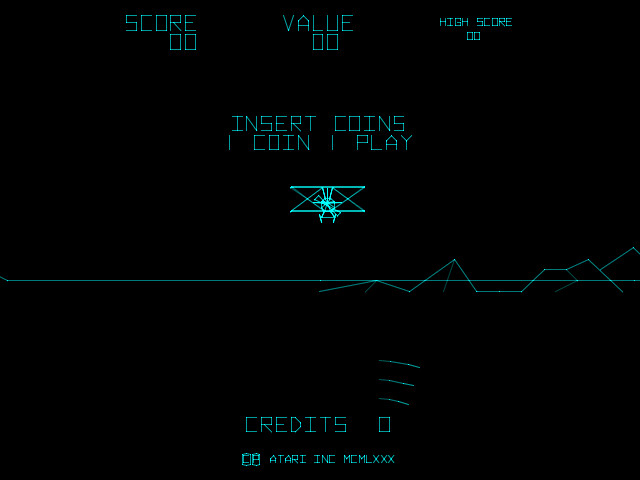This image showcases the minimalist design of an old Atari video game screen, prominently featuring a stark black background. Green neon-like graphics detail various elements. At the top, neatly arranged text shows "Score: 00, Value: 00, High Score: 00." Below this, the center of the screen commands attention with the phrase "Insert Coins, One Coin, One Play" written in matching green text. 

Central to the screen is a simple yet recognizably vintage biplane graphic, giving the impression of aviation from a bygone era. A horizontal line stretches across the screen, simulating the horizon. This line is joined by a jagged, mountain-representing line starting from the middle and moving toward the right, adding a touch of landscape to the minimalist backdrop.

Towards the bottom of the screen, the text "Credits: 0" is displayed alongside the notation "Atari Inc. MCMLXXX," signifying the game's origin and vintage era. Accompanied by a small Atari logo, this setup confirms the game's classic pedigree. The retro aesthetic and simplistic graphics evoke a sense of nostalgia for early video gaming.